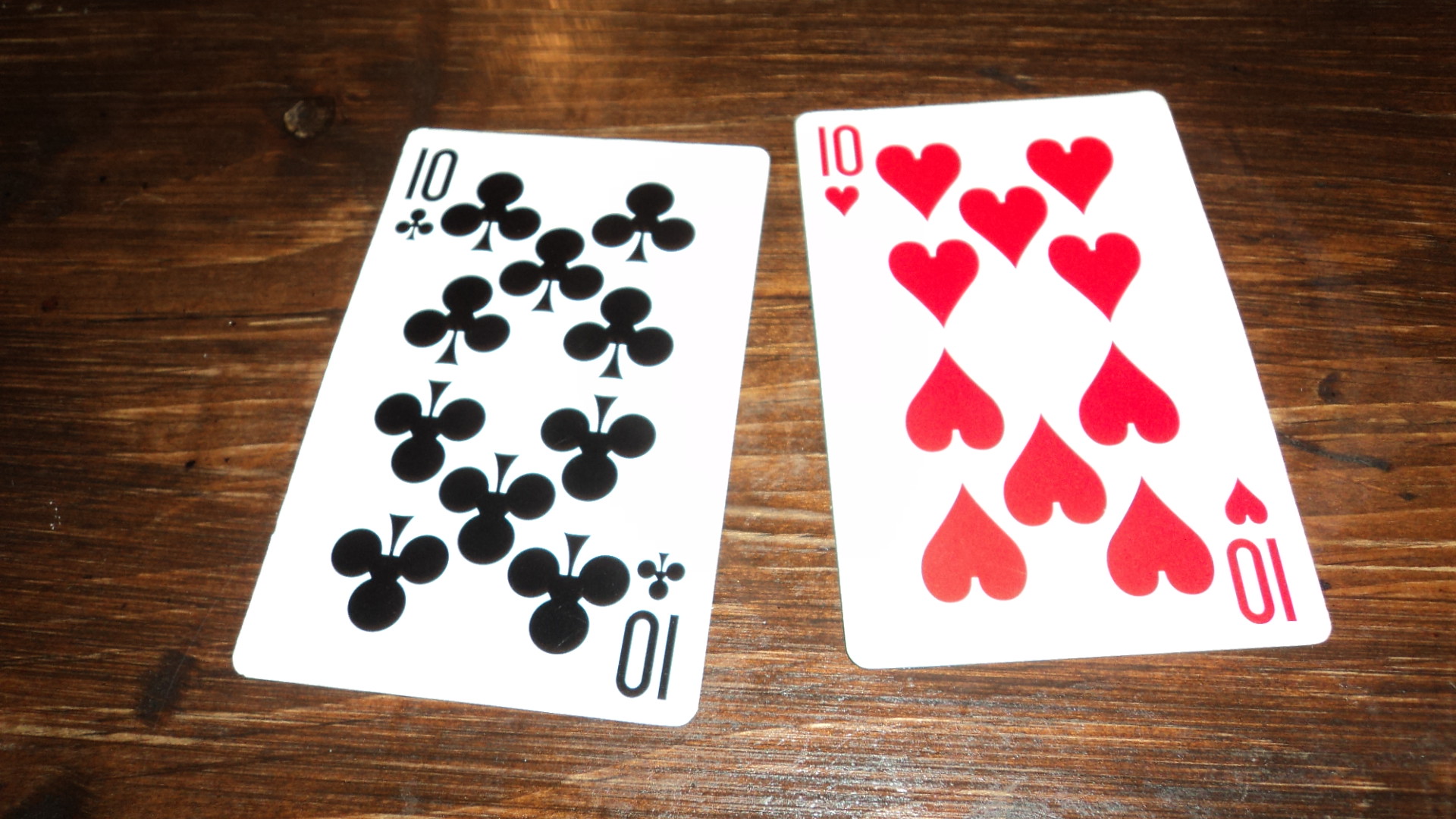This close-up photograph captures two playing cards—the 10 of clubs and the 10 of hearts—laid haphazardly on a rustic wooden table. The cards, positioned slightly askew from each other, prominently display their values and suits, highlighted vividly, likely due to the camera exposure or flash. The table beneath is characterized by its aged, worn texture, featuring a mix of natural grain, scratches, and stains that suggest a long history of use. This old-fashioned wooden surface, with its unintentional flaws and charming imperfections, serves as the sole background, drawing attention solely to the pair of vividly detailed 10s.